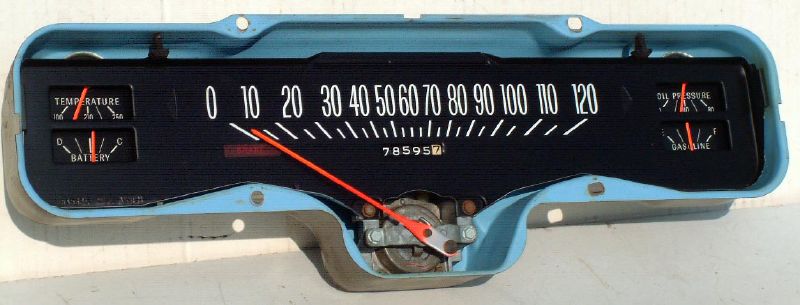This image is a horizontally cropped color photograph focusing on the central dashboard of an antique car. The dashboard, made of light blue metal, spans nearly the entire width of the image, leaving only a small margin on the left and right sides. The centerpiece of the dashboard is an old-fashioned speedometer, prominently displaying white numbers that increment by 10, ranging from 0 to 120. Below the numbers, red gauge lines indicate speed, and the odometer reads 78,595 miles.

On either side of the speedometer, the dashboard features various gauges. To the left, there are two small circular inserts displaying a temperature gauge and another unidentified gauge, both marked with white text and red pointers. Similarly, the right side houses two more gauges in the same white-text-red-pointer style, though these are illegible in the photograph.

The dashboard is secured with visible screw holes along its perimeter, suggesting where it was originally mounted in the car. A noticeable shadow is cast from the dashboard onto a white wall behind it, adding depth to the image. This visually captivating piece is a testament to the vintage craftsmanship of automotive design.